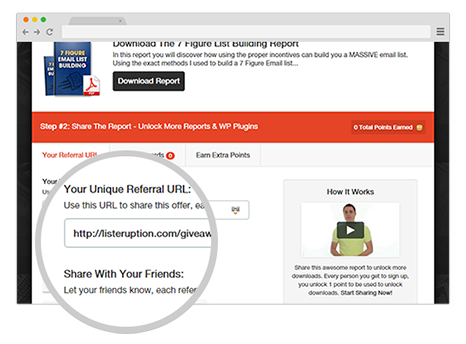The image depicts a Mac screen displaying a promotional message for a downloadable report titled "Download the 7-Figure List Building Report." The text explains that the report will reveal methods for leveraging the right incentives to grow a substantial email list, methods that the author purportedly used to create a 7-figure email list. The next step encourages users to share the report, highlighting that additional reports can be unlocked at "wp-plugins." It provides a unique referral URL, "http://listeruption.com/.giveaway," for users to distribute this offer, with the note to share it with friends to better understand how the process works and unlock further downloads. The layout includes various callouts and action steps emphasizing the importance of sharing the URL to gain extra points and access more resources.